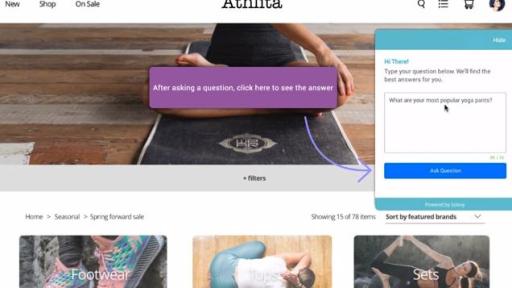This is a screenshot from a website that appears to be named "Athenta," though the name at the top center is partially cut off. In the top-left corner, there are small text links labeled "New," "Shop," and "On Sale." On the top-right side, there are several icons: a magnifying glass for search functionality, a three-line menu icon for navigation tabs, a shopping cart icon, and a person icon for account information.

In the middle of the image, there is a prominent purple box with an instructional message: "After asking a question, click here to see the answer," accompanied by an arrow pointing to the box. The box contains a prompt that reads, "Hi there. Type your question below. We'll find the answers for you." Inside this box, a question has already been typed: "What are your most popular yoga pants?" Below this, there is a clickable button labeled "Ask Question."

Further down the page, there are various clickable categories: 
- The first category is "Footwear," featuring an image of colorful sneakers.
- The second category is not clearly legible, but it shows a woman practicing yoga.
- The third category is "Sets," displaying an image of a woman performing yoga stretches.